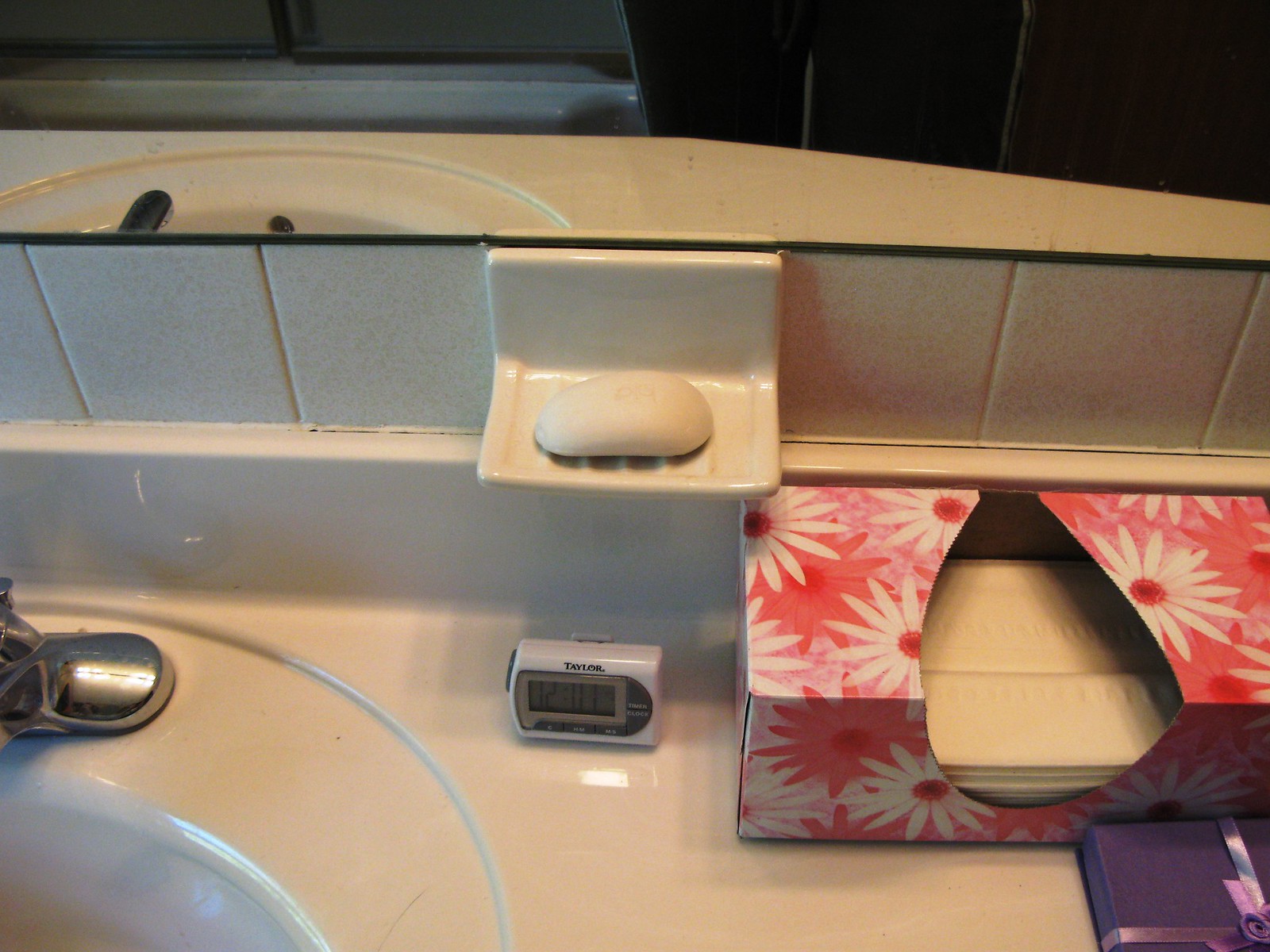A pristine kitchen countertop showcases a myriad of items. At the lower end of the scene, a digital timer displays a time reading of 12. Positioned towards the upper area lies a soap bar, meticulously placed. On the bottom right, an array of napkins accompanied by a pink and white flower arrangement adds a touch of elegance. Adjacent to them, a vibrant purple box stands out. To the left, a sleek sink is present, situated beneath an artfully hung mirror. Above all, gleaming white tiled walls provide a crisp and clean backdrop, enhancing the kitchen's overall neat and organized appearance.